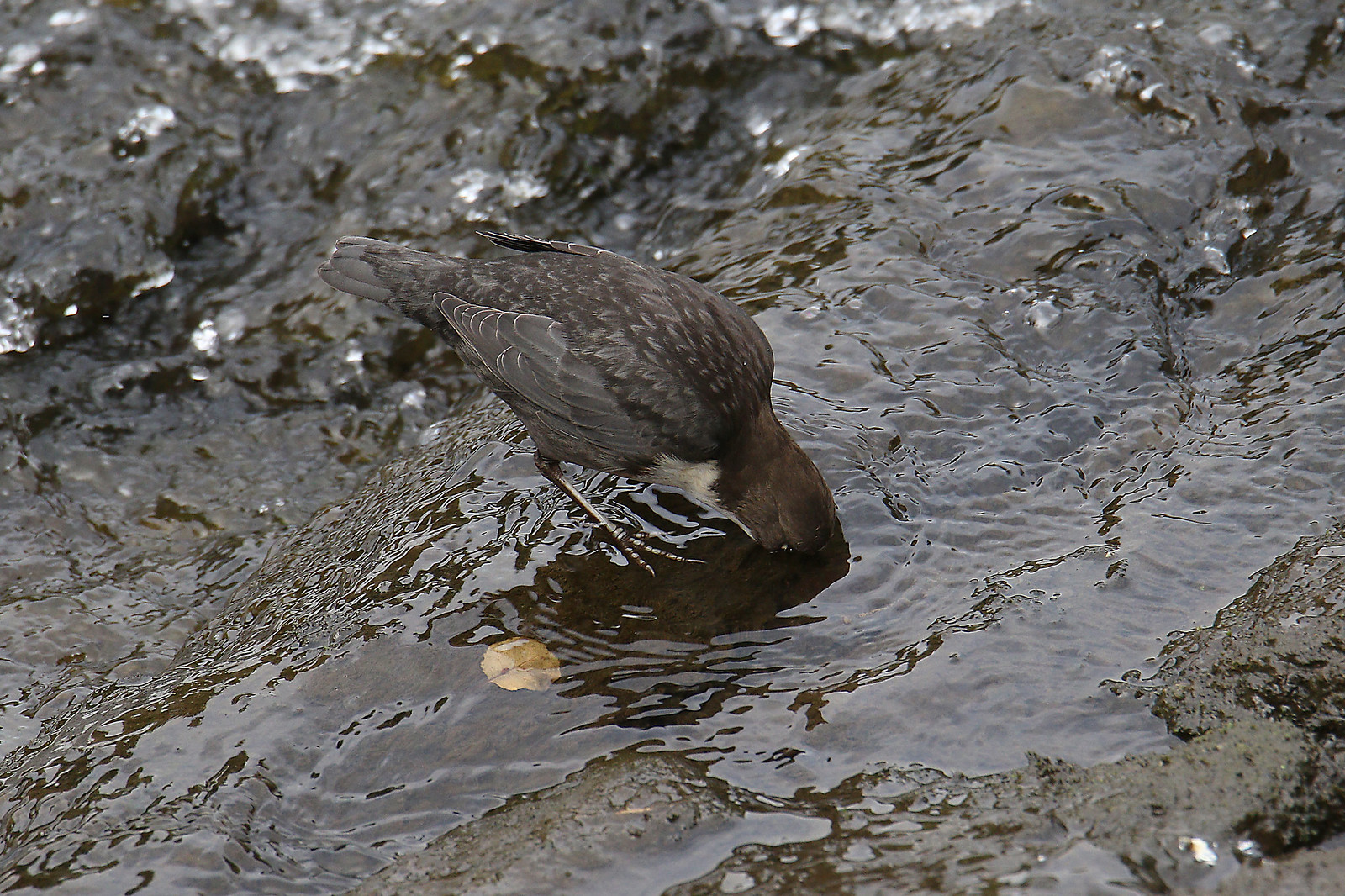In this highly detailed, color photograph taken in landscape orientation, a small bird is at the center, its head bent and partially submerged in a softly flowing creek as it seriously drinks water. The bird, resembling a sandpiper with thin legs, has a dark brown back with light-bordered feathers, a brown head, and a distinguishing white throat and chest. One of its eyes, barely open, is visible just above the water's surface. The transparent creek reveals a golden leaf on the rocky stream bed, indicating the water's clarity. The stream flows diagonally from the top right to the bottom left, contrasting against the brown, muddy background with patches of white near the top of the image, enhancing the naturalistic, photographic realism of the scene.